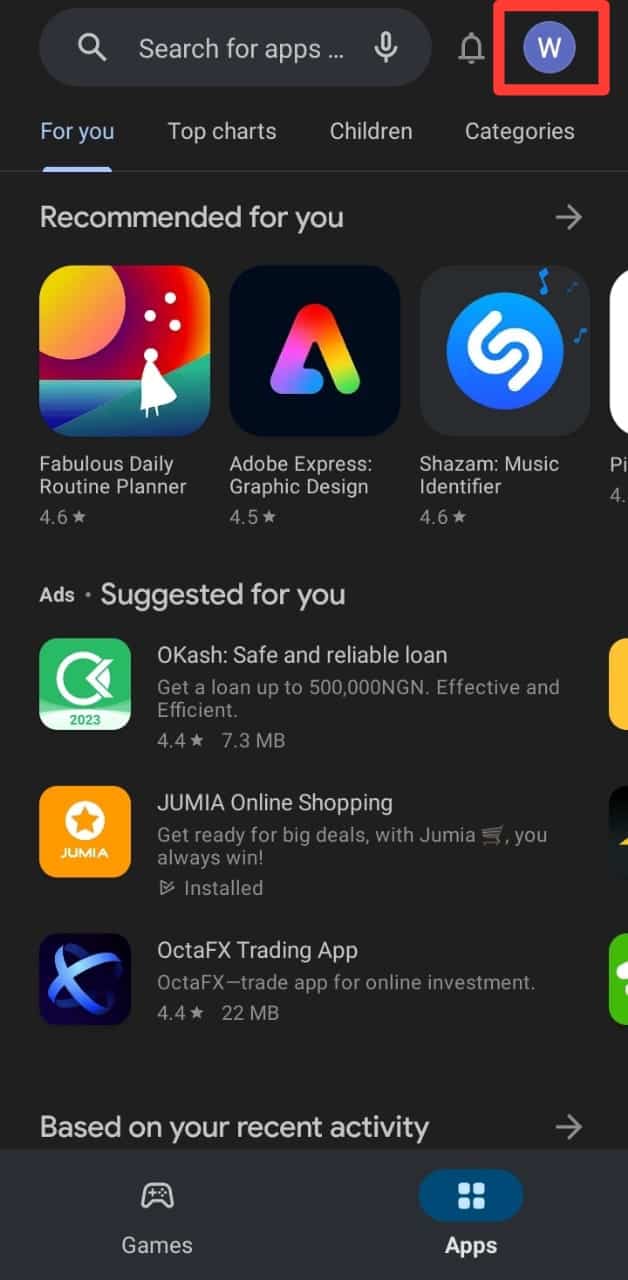This is an image of a mobile or tablet screen displaying an app recommendation webpage with a predominantly black or dark gray background. At the top of the page, there's a search bar labeled "Search for apps." Adjacent to the search bar is a distinctive red box with a black center, featuring a round circle containing a light blue and white "W" icon.

Progressing down the page, the first heading is "For You," followed by "Top Charts" and "Children Categories." Further down, the section titled "Recommended For You" features three prominently displayed app recommendations: 
1. "Fabulous Daily Routine Planner" rated 4.6 stars,
2. "Adobe Express" rated 4.5 stars,
3. "Shazam Music Identifier" rated 4.6 stars.
Each app recommendation includes a small thumbnail image of the app’s logo.

Below this section, there is a heading labeled "Ads, Suggested For You," showcasing three more apps:
1. "Ocash" rated 4.4 stars,
2. "Jumia," marked as "Installed",
3. "OktaFX" rated 4.4 stars.
Each app here is also accompanied by a corresponding thumbnail logo.

The next section is titled "Based on Your Recent Activity." At the bottom of the page, a slightly different colored bar is visible, featuring two tabs: "Games" on the left and "Apps" on the right.